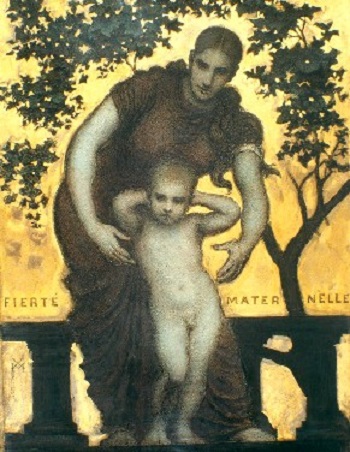The image features a Renaissance-style painting with a golden-yellow background, reminiscent of sunlight either rising or setting. Dominating the scene is a woman of European descent, dressed in a long, brown robe with short sleeves, her hair parted in the middle and neatly pulled back. She is bending forward at the waist, reaching out toward a nude young boy who stands before her. The boy, identified as male, has light brown hair and is striking a peculiar pose with his hands clasped behind his head and elbows out, his right leg extended forward.

Set against this maternal interaction is a backdrop of lush green leaves and tree branches, framing the tender moment between mother and child. The woman stands in front of a black, short, stone railing wall, further accented by black marble columns visible in the background. Text in bold letters stretches across the upper part of the image, spelling "FIERTÈ MATERNELLE," which translates to "Maternal Pride." The intricate details and atmospheric elements combine to evoke a timeless portrayal of maternal care and affection.